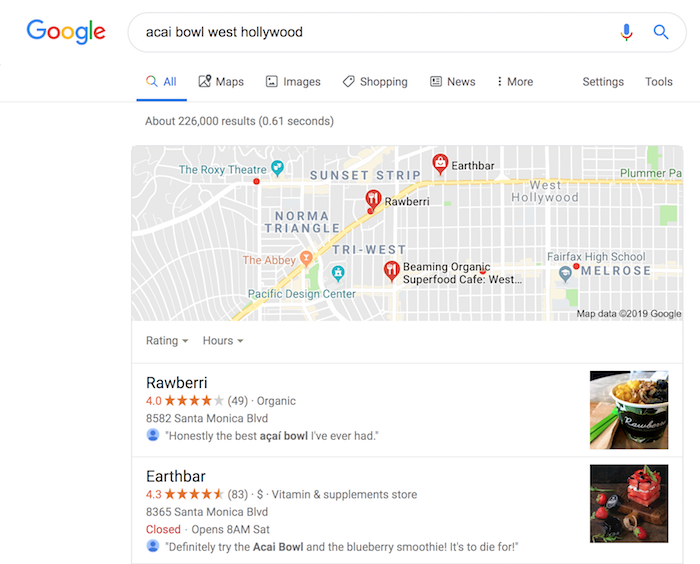This image showcases a Google search results page for "Acai Bowl West Hollywood." In the top left corner, the iconic Google logo features: the letter "G" in blue, the first "o" in red, the second "o" in yellow, the "g" in blue, the "l" in green, and the "e" in red. The search bar displays the query "Acai Bowl West Hollywood," accompanied by a microphone symbol and a magnifying glass icon to the right.

Beneath the search bar, a series of tabs appear, including "All," "Maps," "Images," "Shopping," "News," "More," "Settings," and "Tools," with the "All" tab being selected. A magnifying glass icon also appears to the left of the "All" tab.

Below these tabs, there is a map centered on the Norma Triangle area of West Hollywood. Various landmarks are visible, such as Fairfax High School, Melrose Avenue, the Sunset Strip, the Roxy Theater, and the Pacific Design Center. The map is marked with pins indicating the locations of different acai bowl places in West Hollywood.

Highlighted on the map are two locations. The first is "Rawberry," located at 8582 Santa Monica Boulevard. It boasts a rating of 4 out of 5 stars based on 49 reviews, and a comment praises it as "honestly the best acai bowl I've ever had." The second location is "Earth Bar," situated at 8365 Santa Monica Boulevard. It has a higher rating of 4.3 out of 5 stars from 83 reviews. Despite being currently closed, with a note stating it opens on Saturday at 8 a.m., one enthusiastic review recommends "definitely try the acai bowl and blueberry smoothie. It's to die for."